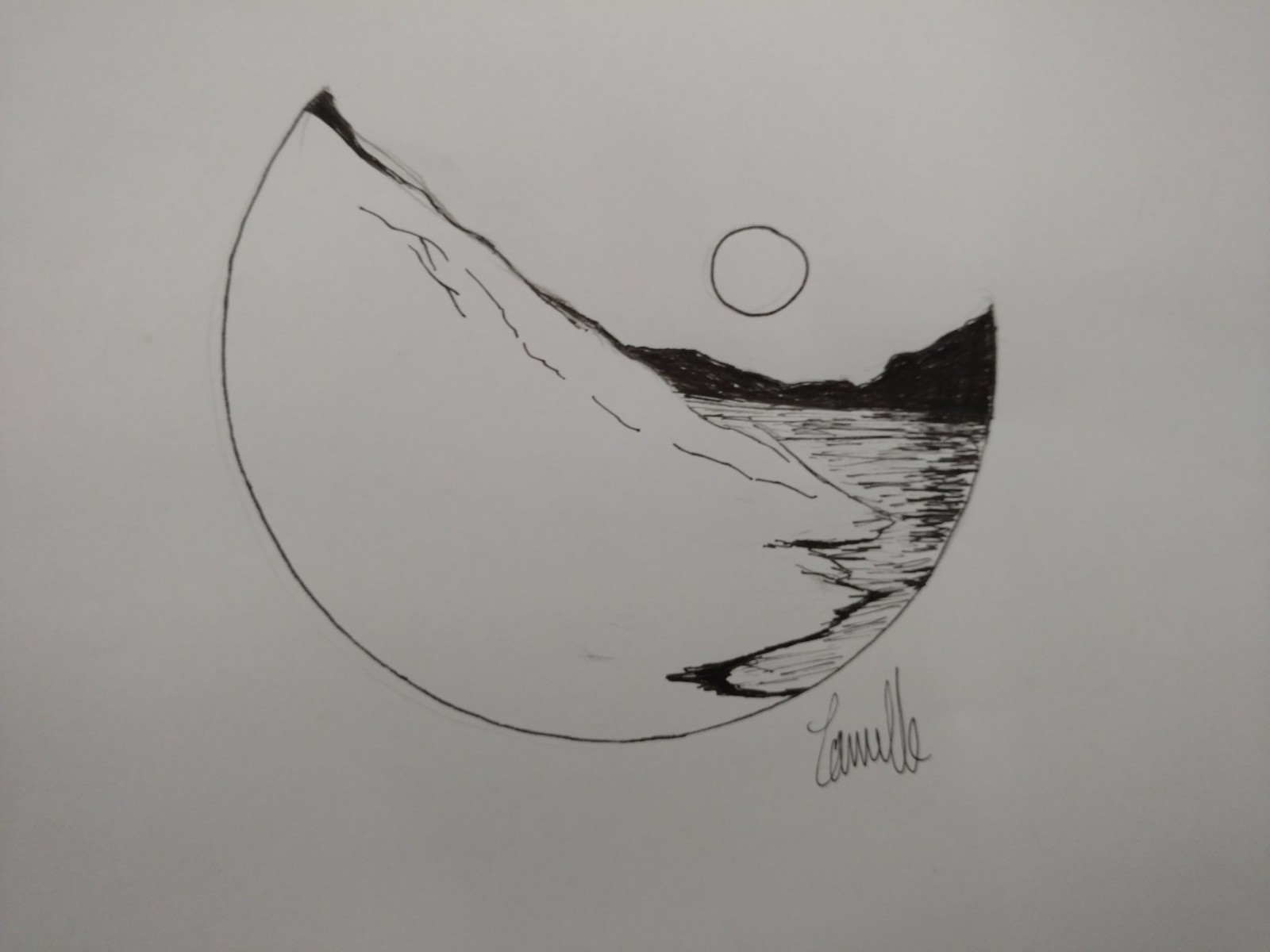The image appears to be a meticulously hand-drawn black and white sketch on smooth, dull white drawing paper portraying a unique and abstract landscape. The central focus is a broken, crescent-shaped form resembling a shattered moon or planet, with its jagged edges intricately rendering depth and texture. This crescent structure, predominantly white with detailed line work, suggests the image of a steep hill descending into the shore of a lake. The water within this lake is illustrated with squiggly lines to convey rippling movement and is sporadically darkened to enhance its texture. On the upper-right portion of the drawing, a series of darkly shaded mountains creates a stark contrast against the lighter hill and lake. Above these dark mountains, a small, uneven circle, possibly representing a sun or moon, hovers in the sky. At the bottom of the image, likely on the right-hand side, there is a barely legible cursive signature that seems to spell "Camille," presumably the artist's name.